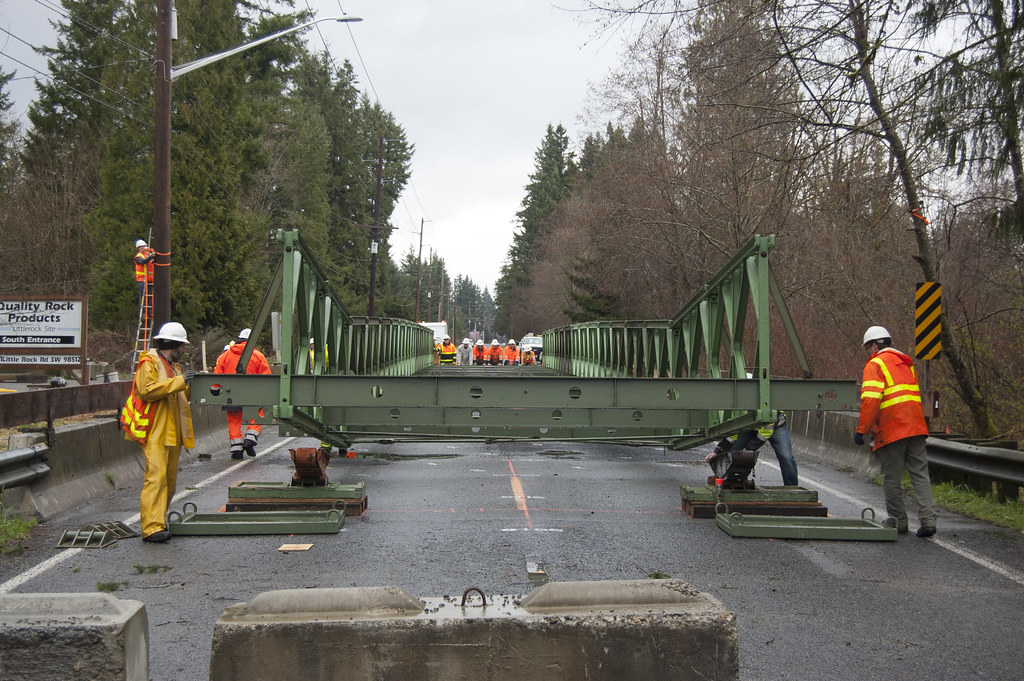This photograph captures a detailed scene of a road construction site where workers are installing a green metal bridge, which appears brand-new and rust-free, likely as a replacement for a previous structure. The road, consisting of two lanes and currently wet from recent rain, features concrete blocks in the foreground to prevent vehicle entry. The workers, adhering to safety protocols, are clad in bright, neon-colored jackets and vests with reflective striping, complemented by white hard hats. On the right, a worker is visible in a bright orange jacket with yellow striping, while another on the left dons yellow attire with an orange vest. Additionally, a person in complete orange gear is walking away on the left side of the image.

The scene includes an elaborate green barrier wall that separates the construction components on either side of the road. Surrounding the construction site, two rows of trees form a natural border, with green foliage on the left and predominantly brown, withered leaves on the right, indicative of the seasonal contrast. In the background, a business sign reads "Quality Rock Products, Little Rock Site, south entrance, Little Rock Road, southwest, 98512," suggesting the location could be within zip codes found in Oregon or California. The cloudy, sunless sky further highlights the overcast weather conditions.